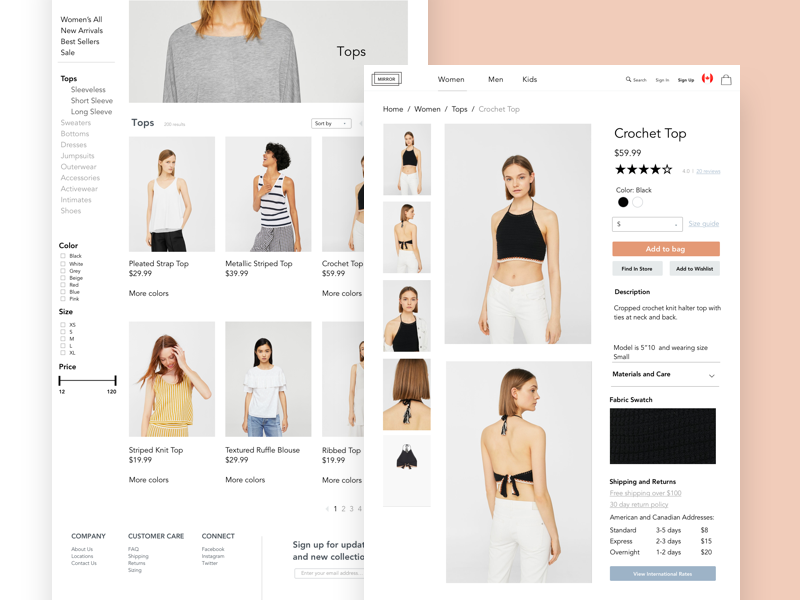This image is a composite screenshot from a clothing website named "Mirror." The left section of the screenshot is slightly longer than the right, featuring a section focused solely on women's fashion. This part of the site showcases various female models donning different outfits, indicating a specific focus on women's clothing.

The header of the page in the left screenshot includes section tabs for "Women," "Men," and "Kids," which implies that the website offers apparel for multiple demographics, though the current view is dedicated to women's clothing. The company's logo, located at the top left, prominently displays two stacked mirror icons and the name "Mirror," which has a visually appealing design resembling layered, forward-facing mirrors or pieces of paper.

The right section of the screenshot details a product listing for a crochet top priced at $59.99. The item has received a favorable rating of 4 out of 5 stars based on 20 reviews. The displayed color of the top is black, but there's an option for a white variant as well. Below the color selection, there's a size guide provided alongside the option to choose different sizes, each possibly having a distinct price associated with it.

This screenshot provides a clear and comprehensive view of the shopping experience on the Mirror website, focusing on a stylish women's crochet top while highlighting the available colors, sizes, and customer feedback.